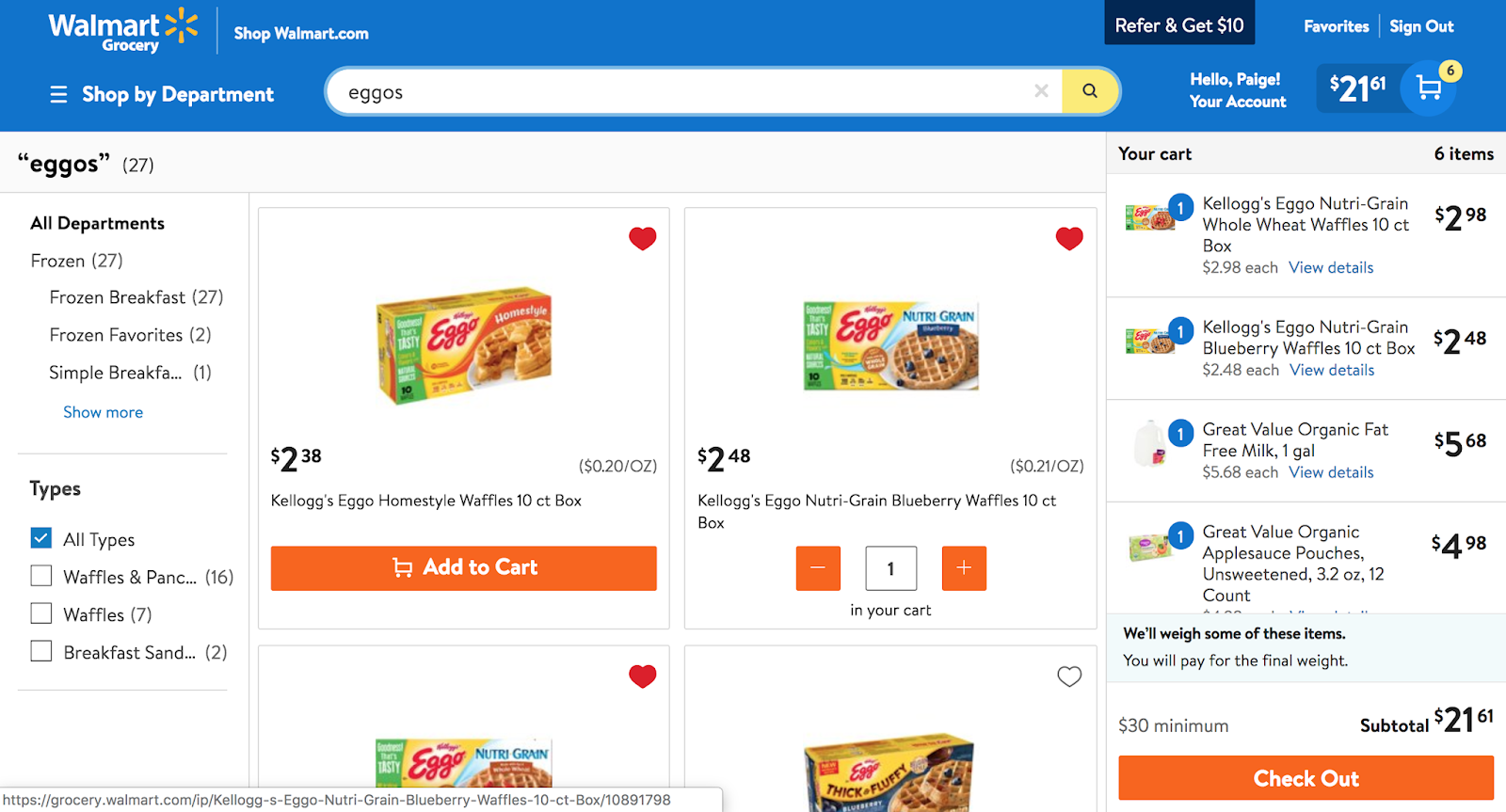**Detailed Caption:**

The image is a screenshot of a Walmart online shopping page for Eggo products. At the top, the Walmart Grocery logo is displayed alongside a search bar with the term "Eggos" entered. The account section shows "Hello, [User's Name]" and indicates that there are six items in the cart, totaling $21.61. Options to view "Favorites" and "Sign Out" are also visible.

The page title reads "Eggos - 27 results," with filter options on the left allowing users to refine their search by department. These departments include:
- Frozen: 27 items
- Frozen Breakfast: 27 items
- Frozen Favorites: 2 items
- Simple Breakfast: 1 item

The search results include various types of breakfast items such as waffles, pancakes, and breakfast sandwiches. The first product listing is for Kellogg's Eggo Homestyle Waffles, available in a 10-count box priced at $2.38, which equates to 20 cents per ounce. The product image features a heart icon, indicating it has been favorited.

Another listed product is the Kellogg's Eggo Nutri-Grain Whole Wheat Waffles, also favorited, priced at $2.48 for a 10-count box.

On the right side of the page, the cart summary details the items currently in the cart:
1. Eggo Nutri-Grain Whole Wheat Waffles
2. Eggo Nutri-Grain Blueberry Waffles
3. Great Value Organic 2% Reduced Fat Milk, one gallon
4. Great Value Organic Unsweetened Applesauce Pouches

The subtotal for the items is $21.61, noting a $30 minimum for checkout. An orange "Checkout" button is prominently displayed at the bottom, indicating that the user still needs to add a few more items to meet the minimum purchase requirement for checkout.